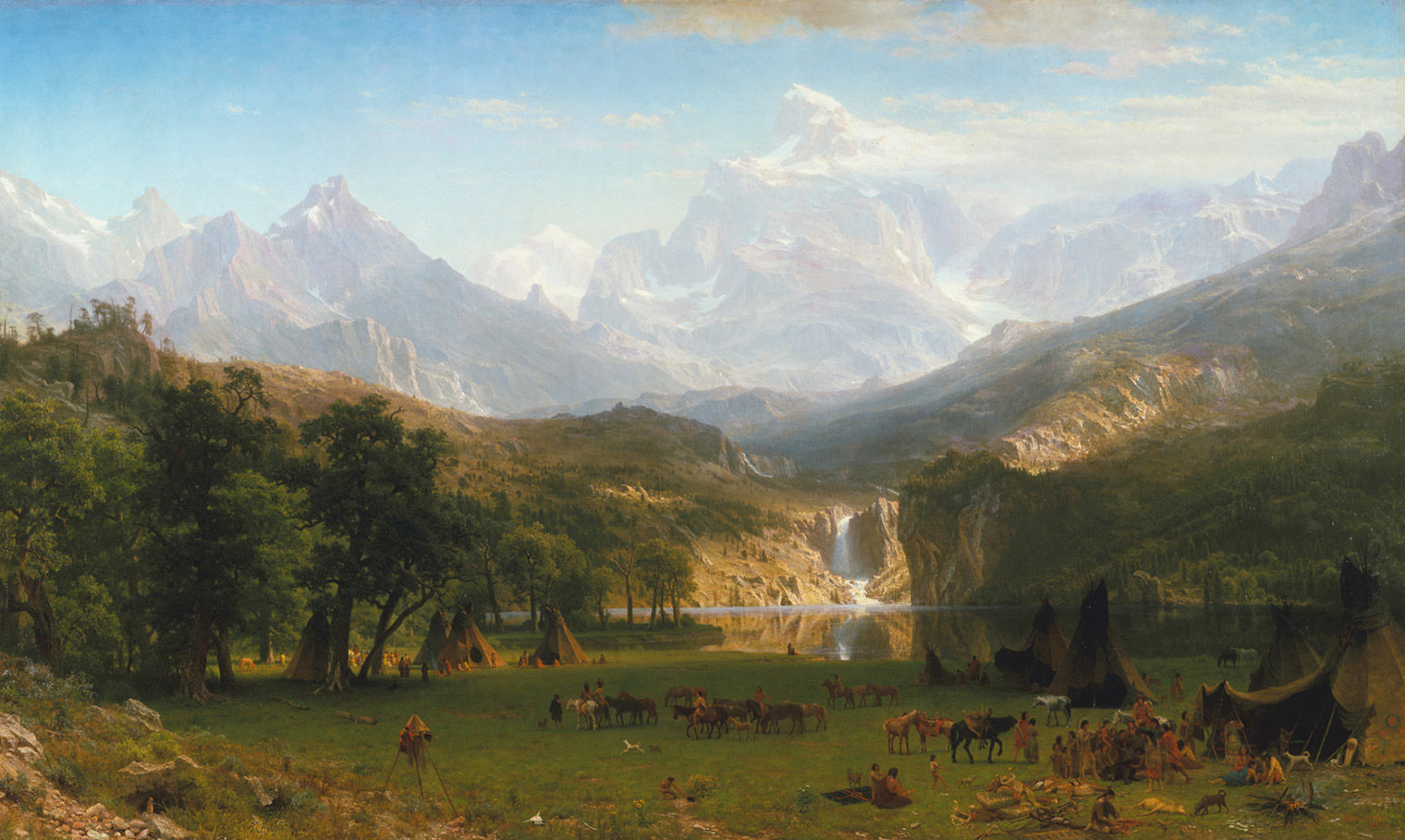The image depicts an expansive, hazy landscape reminiscent of a Hudson River School painting. The top portion features a blue sky interspersed with white clouds, turning into a gray, smoky midsection that accentuates the misty atmosphere. Below, the land transitions into a mossy green-yellow terrain, dotted with dirty mustard-yellow and brown hues, giving off an overall unsightly appearance. At the very bottom, a flat, green-yellow grassy area stretches out, surrounded by patches of black-brown and green canopy-like formations, indicating a forested area.

Amidst this scenery, a group of people and a plethora of horses, along with a few dogs, can be spotted engaging in various activities. There are also numerous dark-colored trees and several teepees, suggesting a makeshift settlement or campsite. These elements contribute to a sense of human and animal activity within this natural setting.

Further back, the landscape ascends into hills and rugged terrain that continue the earthy brown and green color palette. A prominent body of water, possibly a lake, glistens with a waterfall cascading into it, centralizing the composition. The left side of the image is particularly populated with trees and tents, and is bustling with cattle, birds, and people—both children and adults—gathered around.

In the far background, towering rocky mountains capped with sporadic patches of snow rise majestically, completing the vista. The overall scene, although cloudy and smoky at points, is brightly lit and vividly colored, capturing a dynamic and bustling outdoor setting framed by natural grandeur.